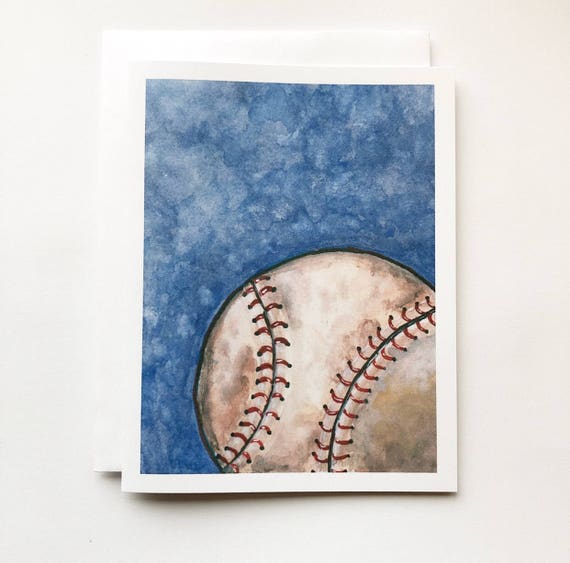The image displays a watercolor painting of a baseball, placed on a white surface. The artwork, approximately the size of a piece of printer paper or slightly larger, features a baseball as its focal point, occupying about half of the painting. The lower right portion of the baseball is cut off. The ball itself is depicted in a dirty, weathered appearance, with a mix of khaki, tan, beige, reddish brown, and gray hues. The traditional red stitching of the baseball is clearly visible. Surrounding the baseball is a denim-blue watercolor background. The entirety of the artwork is slightly skewed and set against a pristine white background.